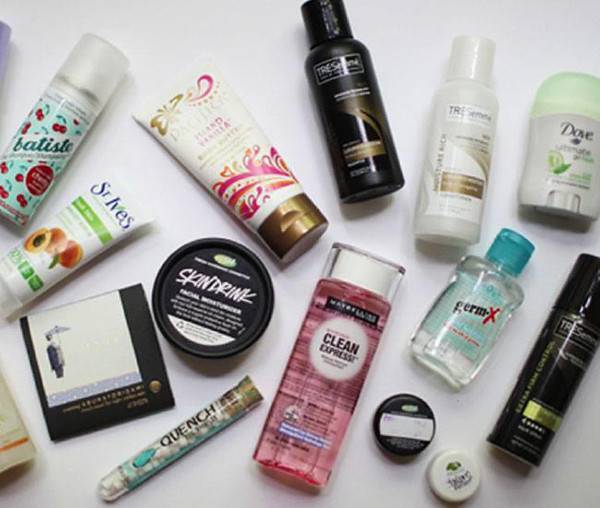This detailed top-down photograph showcases an assortment of 10 to 12 travel-sized beauty, skincare, and hygiene products arranged on a pristine white surface. The items are all laying flat, allowing a clear top-view of their labels and designs.

Starting from the top left, we find:

1. A cylindrical container adorned with a light blue and cherry print design. The label reads "batiste," written in a cursive font, accompanied by a red circle.

2. To the right, there is a hand cream tube labeled "French Vanilla." The container is decorated with pink and gold ornamental patterns, featuring a gold cap that remains attached when opened. Black text is visible on the label.

3. Next is a travel-sized Tresemme conditioner in a black bottle, highlighted by the brand's iconic gold logo.

4. Adjacent to it is a matching Tresemme travel-sized conditioner, this one in a white bottle with gold accents.

5. Following that, we see a small Dove deodorant. The container is predominantly white with light green accents including the cap.

On the second row, from the left:

6. A St. Ives facial scrub container is visible, showcasing a label with an image of peaches, green borders, and white text.

7. Next is a circular container labeled "Skin Drink."

8. A rectangular bottle of "Clean Express," which is see-through, revealing a vibrant pink liquid inside. The bottle is covered in text and has a clear cap.

9. To its right is a clear GermX hand sanitizer featuring a blue cap.

10. There is also a miniature black Tresemme hairspray bottle with the characteristic gold logo.

11. Two small circular containers, possibly lip balms, resembling the size of a quarter and a half dollar, are nestled together. They do not have visible labels.

12. A tube with "Quench" written on it, possibly containing either Q-tips or pills, can be seen.

13. Finally, there is a small black square item with a grainy illustration showing someone holding an umbrella. The image quality is low, making it difficult to decipher the details.

This image provides a comprehensive look at an array of well-loved travel-sized products, perfect for a quick getaway or on-the-go personal care routines.